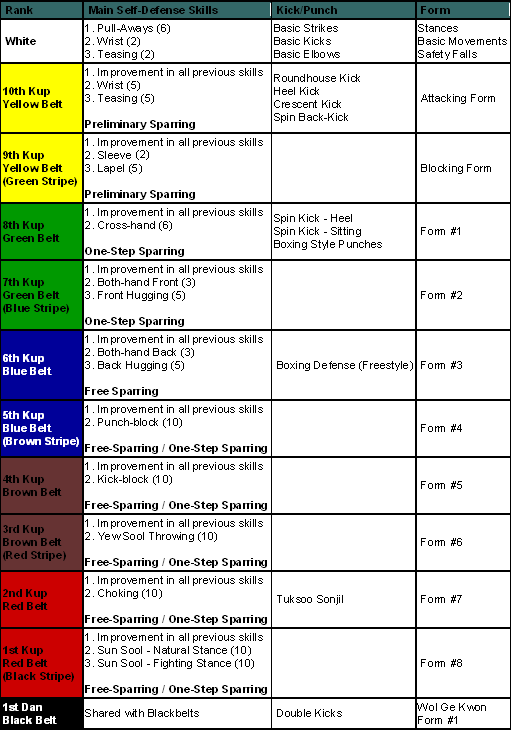The image is a detailed chart with four columns and twelve rows, used for ranking martial arts proficiency levels. The chart visually represents different belt levels and their corresponding skills required to attain each rank. 

- The **first column** is labeled "Rank" and lists the progression from White Belt to Black Belt, including intermediate colors and stripes such as Yellow Belt, Yellow Belt Green Stripe, Green Belt, Green Belt Blue Stripe, Blue Belt, Blue Belt Brown Stripe, Brown Belt, Brown Belt Red Stripe, Red Belt, Red Belt Black Stripe, and Black Belt. 

- The **second column**, titled "Main Self-Defense Skills," includes various skills for each rank. These skills differ as they progress, starting with "Pull Aways," "Wrist," and "Teasing" for the lower belts, and advancing to "Preliminary Sparring" and "One-Step Sparring" for intermediate levels, culminating in "Free Sparring" and "One-Step Sparring" for the higher belts.

- The **third column** is labeled "Kick/Punch" and specifies the proficiency required in these fundamental techniques for each level.

- The **fourth column** named "Form" likely details the forms or patterns that practitioners must master at each belt level.

This grid format provides a comprehensive overview of the martial arts curriculum, categorizing each rank's specific requirements through color-coded squares that match the belt colors. The image serves as a reference for tracking the progression from beginner to advanced levels in martial arts training.